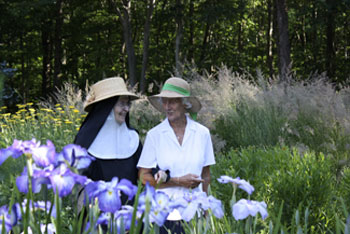In this evocative photograph, two elderly women walk arm in arm through a serene forest, surrounded by tall grasses and vibrant flowers. One woman wears the traditional garb of a nun, complete with a habit and glasses, while the other is dressed in a white shirt, accented with a woven straw bonnet adorned with a green bandana. The women, both smiling and seemingly engaged in a warm conversation, mirror each other with matching bonnet hats. The forest backdrop is painted with the long shadows of late evening, casting a tranquil, ethereal light through the trees. In the foreground, striking violet, white, and yellow lily-like flowers punctuate the scene, adding a burst of color to their peaceful stroll.